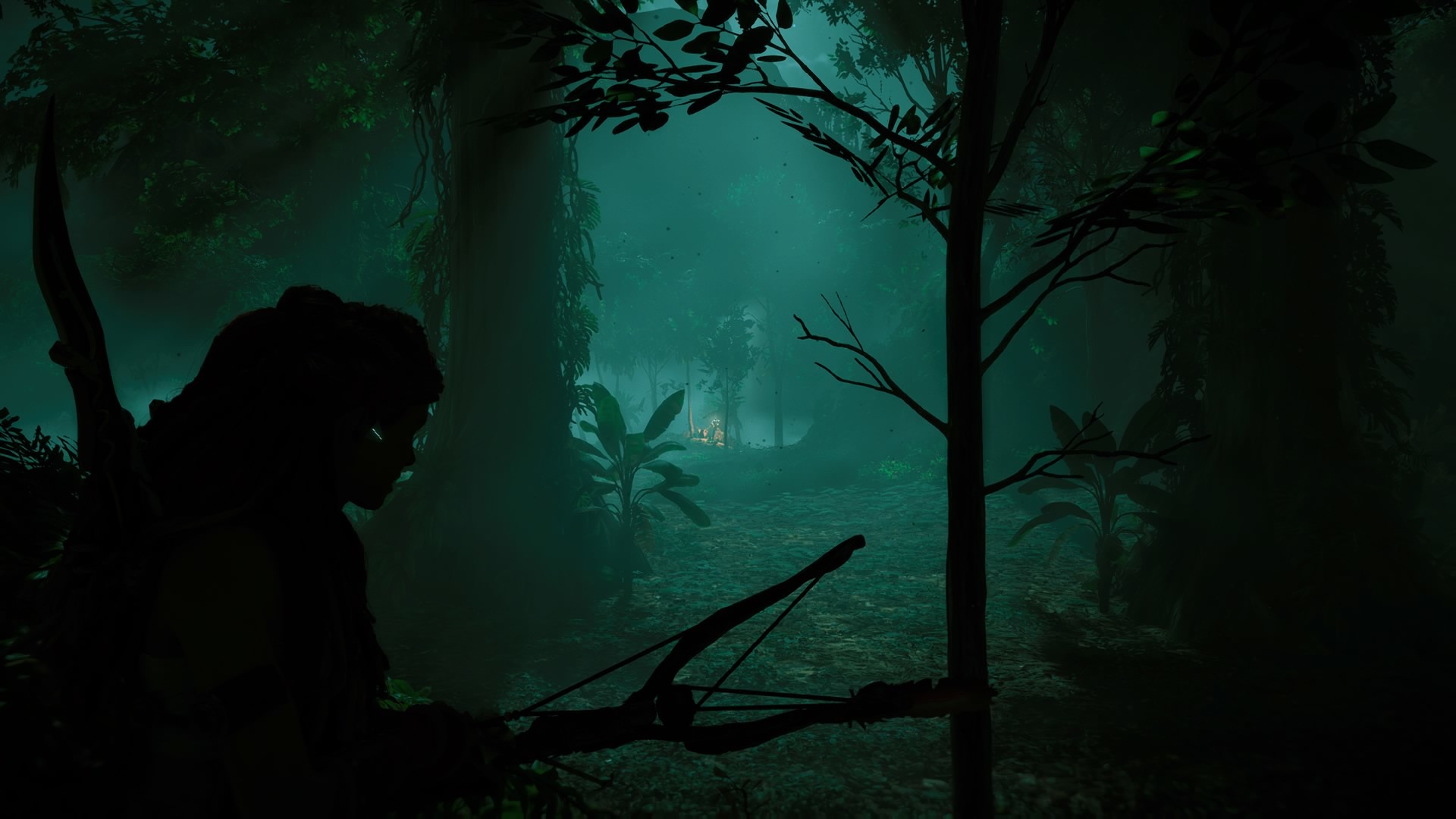This image is a screenshot from a computer-animated video game, giving a distinctly three-dimensional, yet not photorealistic, feel. Bathed in blue-green hues, it portrays a densely wooded forest at evening, shrouded in darkness and fog. A narrow pathway cuts through the trees in the middle of the image, leading into the misty distance. In the foreground, the shadowy figure of a person is visible; this character, likely a soldier or hunter, holds a large slingshot-like tool and carries a bow for arrows on their back. Their features are obscured by darkness, making them appear as a silhouette. The scene exudes an ominous and mysterious atmosphere, with patches of lighter blue-green suggesting possible reflections, perhaps from a pond, and indistinct shadows that add to the eerie feeling of uncertainty about whether they are trees or other figures.